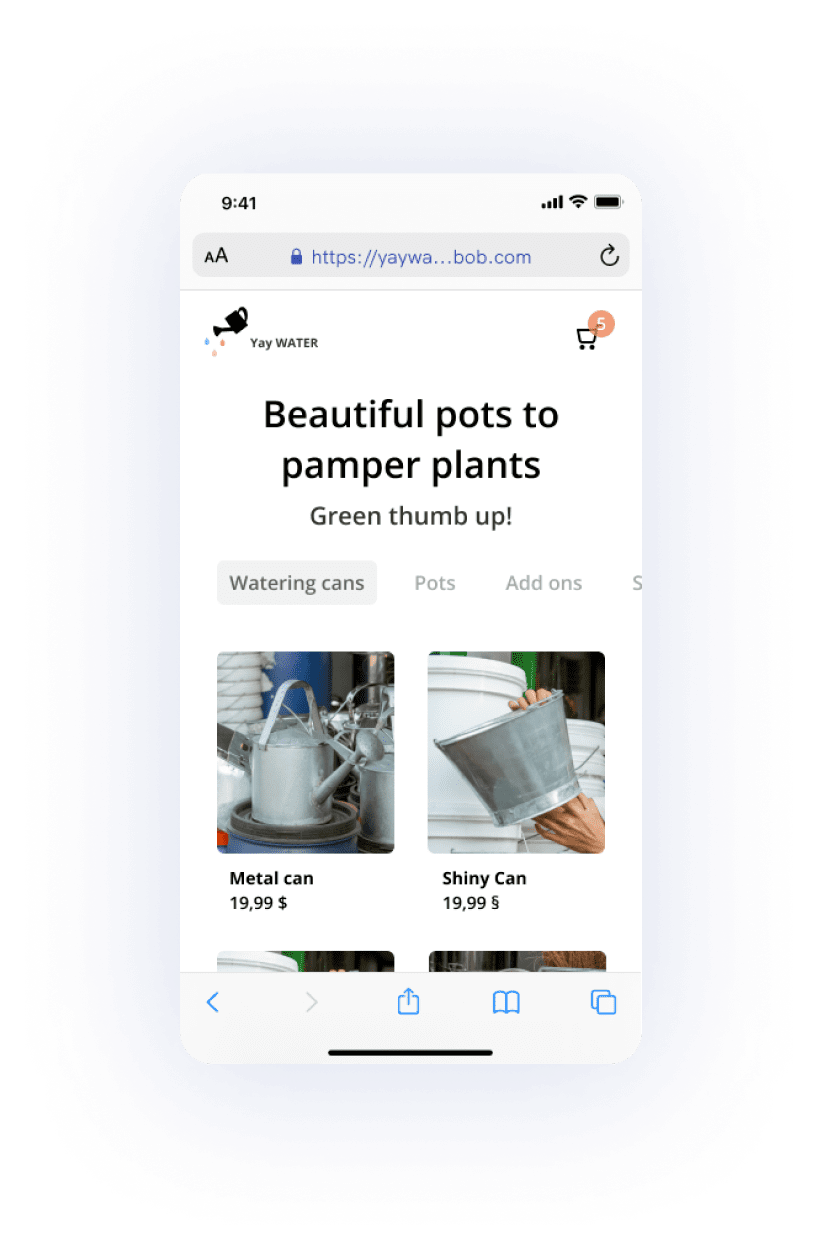Screenshot Caption: 

This image captures a screenshot of a smartphone displaying a shopping page from the website "Yay Water," notable for its logo, which features a watering can. The URL partially shown at the top ends in "bob.com." On the right top side of the interface, a cart icon indicates that the user has five items added to their cart. The page is titled "Beautiful Pots to Pamper Plants" with a subheading that reads "Green thumb up." 

Highlighted in the subcategories is the "Watering Cans" section, showcasing two distinct products along with their images and prices. The first item is labeled "Metal Can," priced at $19.99, resembling a typical outdoor watering can. The second item, also priced at $19.99, is called "Shiny Can." However, this item is notable for lacking a spout and handle, more closely resembling a standard container. The page suggests additional options to be revealed through further scrolling.